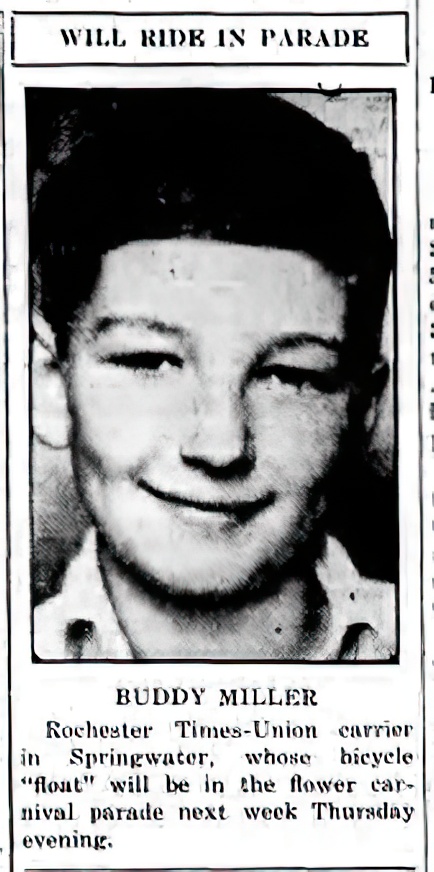This black-and-white image appears to be a cropped snippet from an old newspaper, featuring a center-aligned photograph of a young boy, likely a teenager, positioned prominently. Above the photo, within a white box bordered in black, the headline reads, "We'll Ride in Parade." The boy, identified as Buddy Miller, has black hair and is dressed in a white collared shirt, smiling directly at the camera. This image evokes the feel of a school yearbook photo. Below the photo, the brief caption in all caps reads, "Buddy Miller," followed by a slightly distorted text: "Rochester Times Union carrier in Springwater, whose bicycle 'float' will be in the Flower Carnival Parade next Thursday evening." The black and white hues, along with varying shades of gray, contribute to the historical aesthetic of the clipping. Partial letters are visible on the right side, indicating the snippet has been cropped from a larger page.